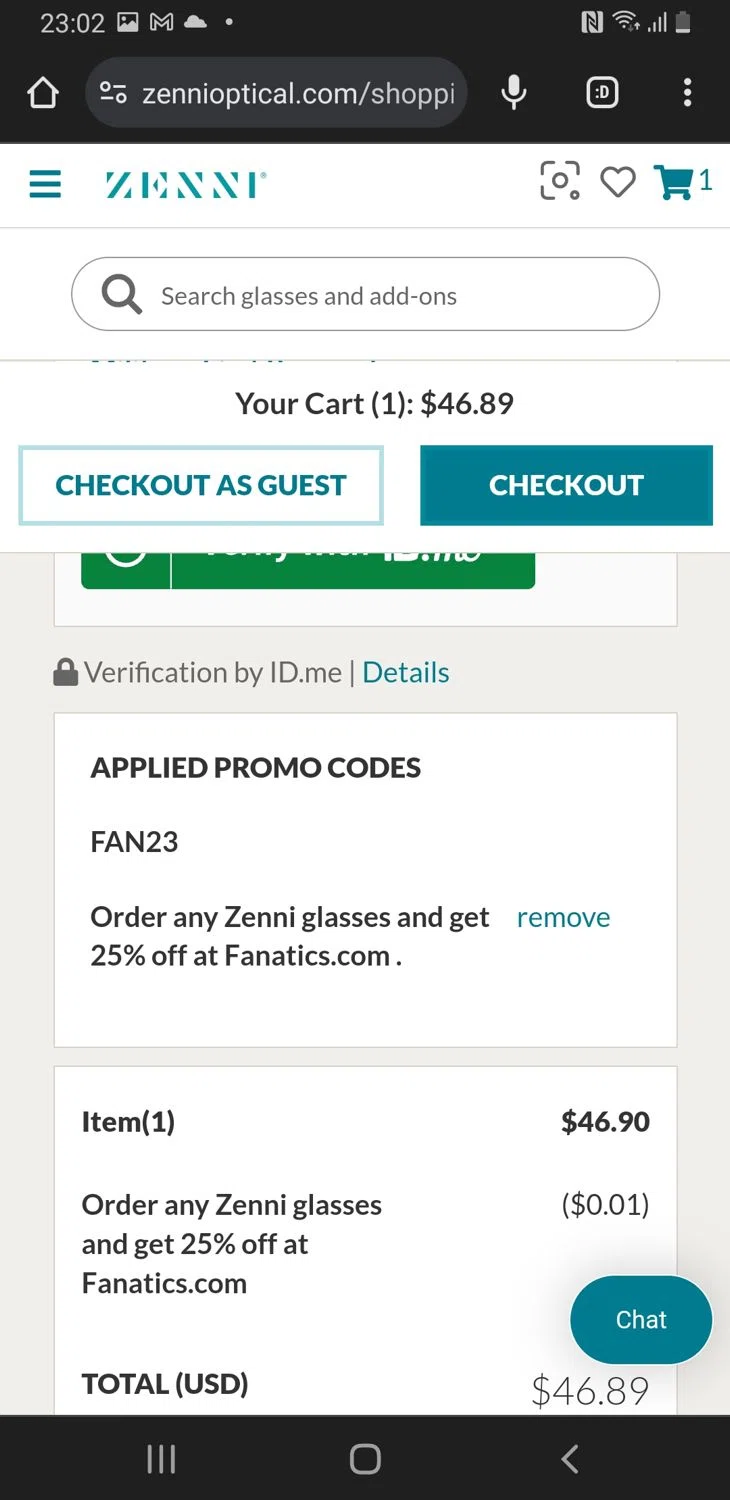This image captures a screenshot of the zinnioptical.com website as viewed on a mobile device. Dominating the upper portion of the screen is the Zinni Optical banner, immediately followed by a prominent search bar with the placeholder text "Search glasses and add-ons". The main focus of the page is the checkout cart, which details a pair of glasses priced at $46.90. A promo code, "fan23", has been applied, offering a 25% discount associated with fanatics.com. Highlighted options at the top of the cart allow the user to either "Checkout as Guest" or "Checkout and Log In". Notably, due to the promo code, the new total for the cart is adjusted down slightly to $46.89.